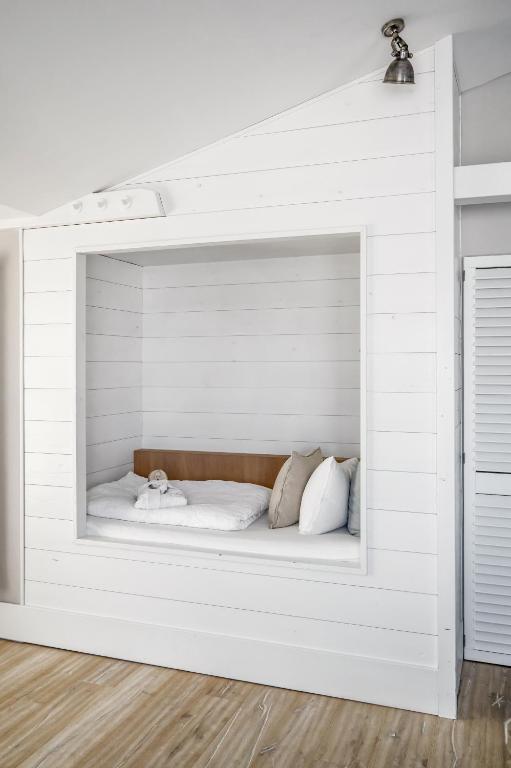The photograph captures an indoor room illuminated by natural light, possibly an attic space due to its inclined white ceiling extending from the upper left to the upper right corner. The dominant feature is a wall with horizontal white wooden slats and a recessed square nook at its center. This cozy nook, framed in the same white paint as the surrounding wall, houses a long rectangular bedroll complemented by a few cushions on the right side and a low dark brown wooden backboard. The bedroll area appears snug, designed more for sitting than sleeping. On the right-hand side of the room, adjacent to this nook, another recessed area is visible, featuring a closed slatted grid door. The floor is comprised of light brown or tan wooden planks, enhancing the room's warm and inviting atmosphere. A stainless steel lamp hangs from the ceiling, though it is not currently lit, adding to the rustic charm of the room.